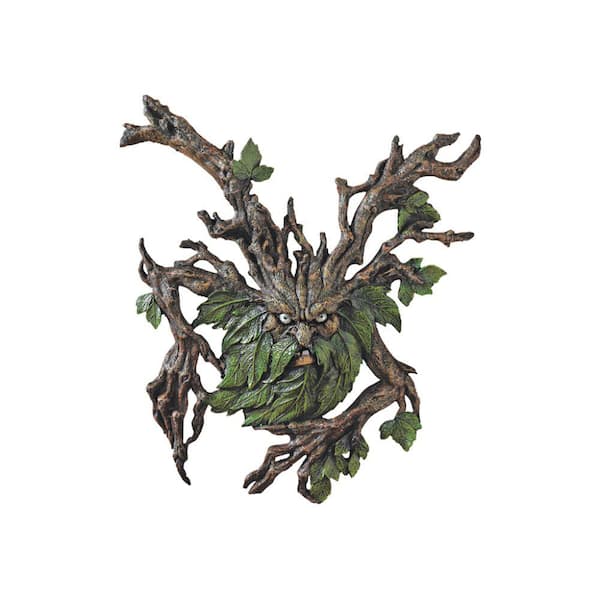This portrait-oriented color photograph showcases a highly detailed 3D wall sculpture designed to resemble a tree-like creature. The sculpture appears to be made of wood or a material fashioned to mimic wood, such as clay. The central figure, portraying an angry or grouchy old man, features a face with distinct, clear eyes, a large nose, and a furrowed brow, creating an intense expression. His facial hair, consisting of a mustache and full beard, is crafted from dark green leaves. The creature's 'hair' also includes leaves on the sides of its head.

Two large, natural-looking branches extend from the top of its head, giving the appearance of horns, with more leaves hanging from them. Long, uneven arms shaped like tree branches extend from its body, and these branch-hands possess a skeletal quality. Some of the leaves also hang from the hands, adding to the organic, forest-like aesthetic. The background of the image is white, making the sculpture appear to float and enhancing the visibility of its intricate details.